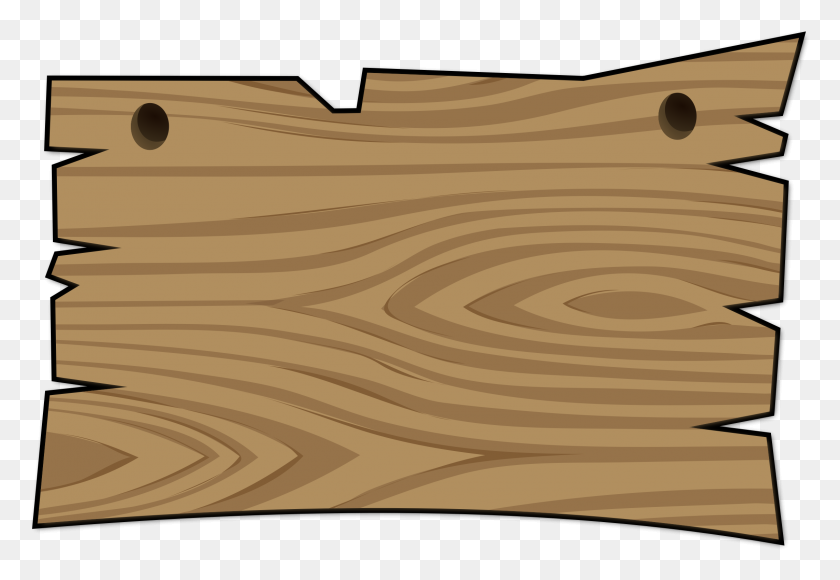The image showcases a cartoon-style illustration of a jagged, misshaped brown wooden board. The uneven edges include V-notches and a prominent notch on the top left. The plank features two black holes towards the top, appearing as though they are drilled in and possibly intended for securing or hanging the board, like a makeshift sign. The wood grain is represented in dark brown against a lighter brown background, highlighting the natural whorls and character of the wood. Encircling the board is a thin black border. The backdrop is a white and gray checkerboard pattern, similar to a Photoshop transparency grid, filling the entire surface area of the image. This detailed rendering captures the rustic and utilitarian essence of the wooden plank, making it suitable for various creative and promotional applications.